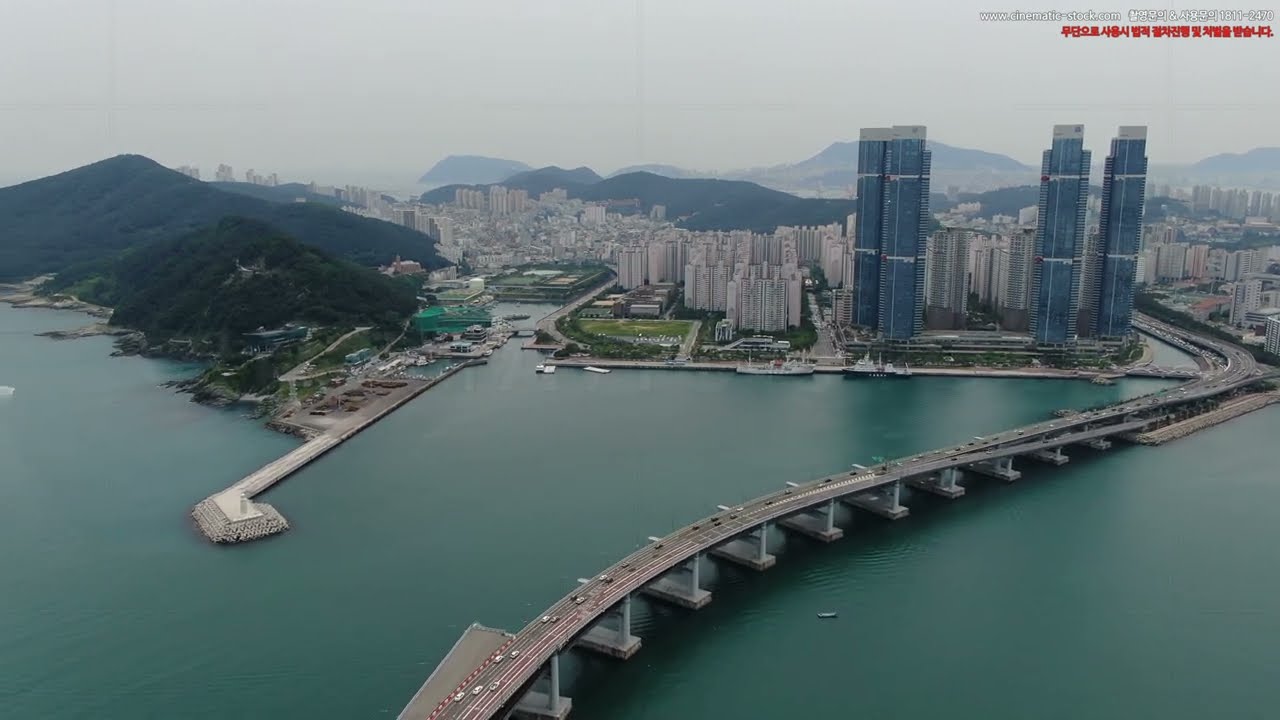The image is an aerial view of a modern coastal city, set in a valley between hills and mountains. Prominent on the right side of the city are four towering skyscrapers made of steel and glass, standing over a cluster of shorter, yet still impressive white and gray stone buildings. To the left side of the image, there are smaller hills or mountains covered with grass and trees. Near these, there's a jetty or dock area, indicating a harbor or bay. The turquoise-green water is exceptionally calm, as still as glass, contributing to the serene atmosphere. A sleek bridge stretches from the center left towards the center right over the water, connecting to the city's road network with tiny cars visible on it. Faded mountains loom in the hazy background, adding depth to the scene. Tiny red and white Korean text is located at the top right corner, indicating the source of the image. Overall, the cityscape appears meticulously organized, almost model-like in its consistency and structure.